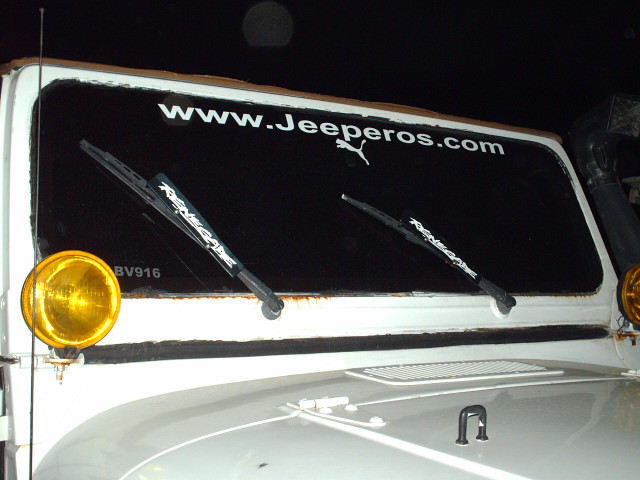In this detailed photograph, the focus is on the front portion of a white Jeep against a completely black background, making the vehicle's features highly visible. The image prominently shows the Jeep's windshield and hood. The windshield is particularly dark, almost black, with the website "www.jeeperos.com" displayed in striking white letters across its top. Directly beneath this text, the iconic Puma logo is also rendered in white. The Jeep's windshield wipers, both in a raised position, are black with white lettering on the arms, possibly indicating the word "Renegade." Just above the hood, there is a gray U-shaped hook with a vent positioned behind it. On both sides of the Jeep's windshield, brightly shining yellow lights are visible, likely serving as turn signals or fog lamps. A noticeable detail includes the inscription "BV916" in white, located near the yellow light on the left side of the vehicle. Additionally, signs of aging are apparent, as rust can be seen around the bottom edge of the windshield frame.